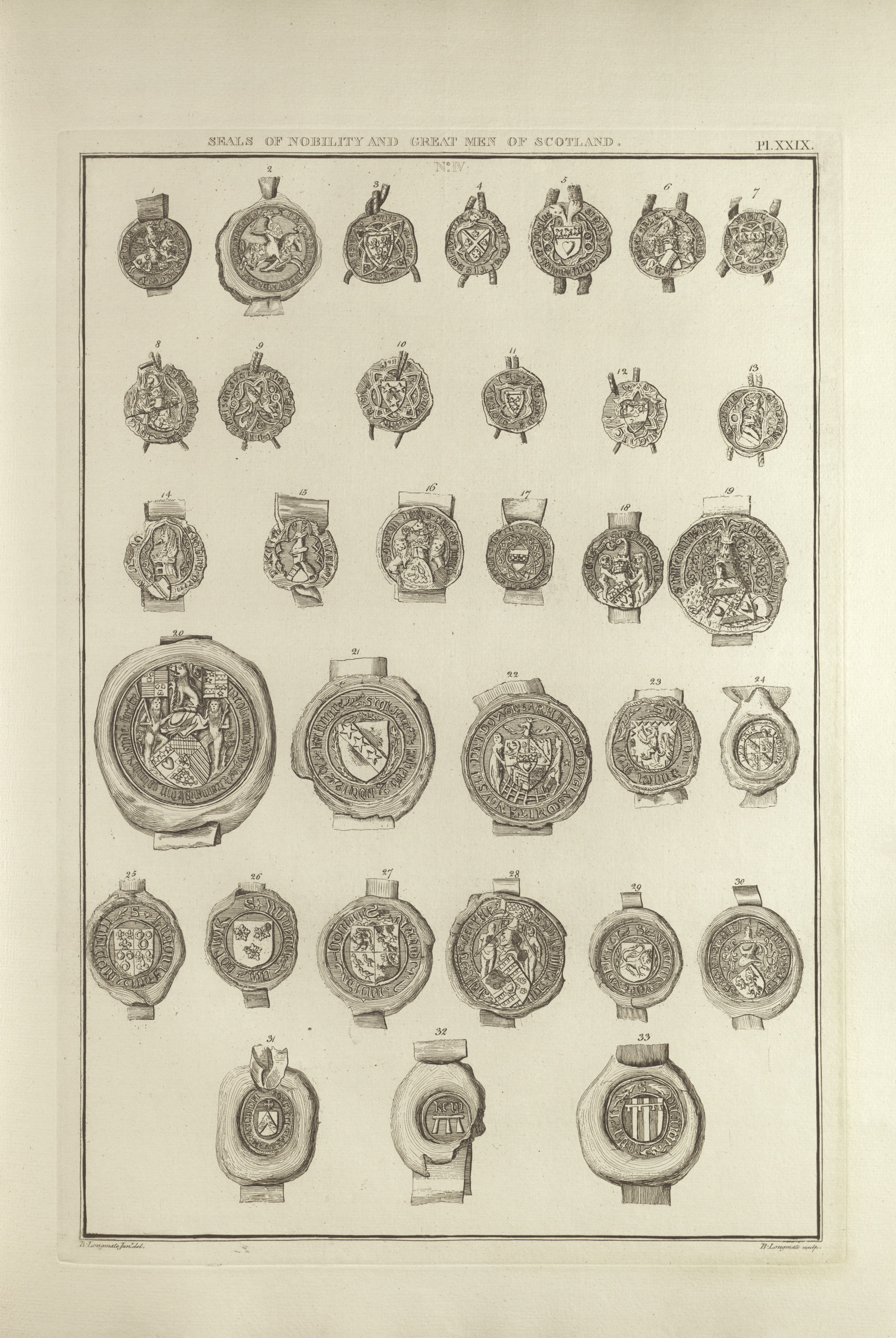The photograph shows an image resembling a historical poster, stuck to a white wall with a white background that blends seamlessly into the wall's color. The image features a black border and includes a somewhat legible title at the top that reads, "Seals of Nobility and Great Men of Scotland," offering a hint about the subject. The picture itself displays numerous rows of seals, historically used for stamping official documents. Detailed in six rows, the top five rows contain at least five seals each, while the bottom row has three, totaling approximately 40 seals. Each seal is distinct, featuring varied designs such as a man on horseback, a knight on horseback, shields with different emblems like four-leaf plants, a heart, and three stars. The seals are meticulously ornate, evoking the historical wax stamps seen in olden days, and the page they are presented on is a beige color, suggesting it might be from an ancient book or document, likely suitable for display in a museum.